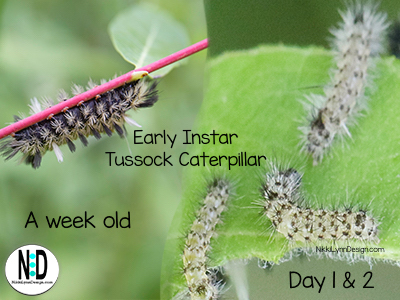The poster titled "Early Instar Tussock Caterpillar Development" presents a detailed and modern visual documentation of a caterpillar's growth stages against a muted green leafy background. The progression from day one and two to a week old is clearly depicted. The caterpillar in its early stages is shown as a light brown creature with fluffy, white hairs. As it grows to a week old, it becomes a bit darker and possibly more fuzzy. The image features four caterpillars at various stages: three on the right side at days one and two, and one on the left showcasing its week-old appearance. Notably, one caterpillar is pictured inching along a vivid hot pink stem. The bottom left of the poster includes a logo resembling a white circle with black block letters "ND" and three turquoise circles in between, which transition in shade from light to dark. Below this logo is a partially legible URL, likely "nicklyndesign.com", referring to the source of the poster.